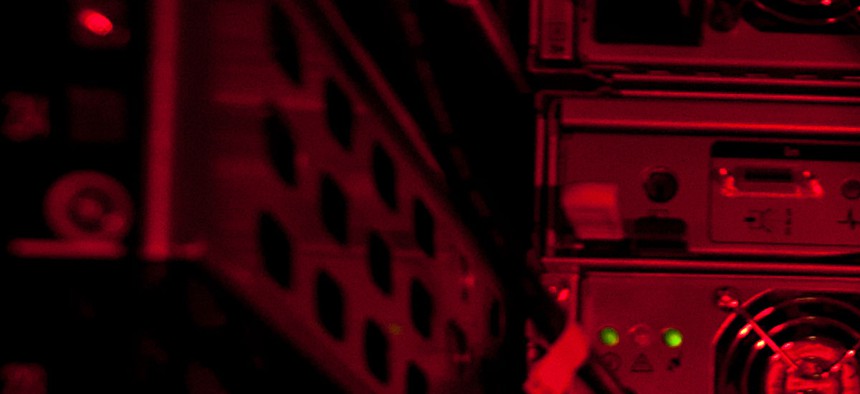This image, heavily bathed in red illumination, appears to be a close-up of a complex piece of machinery or technology, potentially from a server room or the interior of a powerful computer. The red light lends an almost sci-fi aesthetic to the scene. Dominating the bottom right-hand corner is a fan, which suggests some kind of cooling component typical of electronics. The environment is metallic, with a connection port visible on the right that might be intended for a computer monitor. This port is flanked by two lit green lights, with an unlit space between them. The surroundings are visually crowded, making it difficult to discern specific details. On the left side of the image, there is a metallic grid or grate, possibly designed for ventilation, with approximately 12 to 14 openings. The overall structure includes various rectangular shapes and air holes, adding to the abstract nature of the red-and-black design.